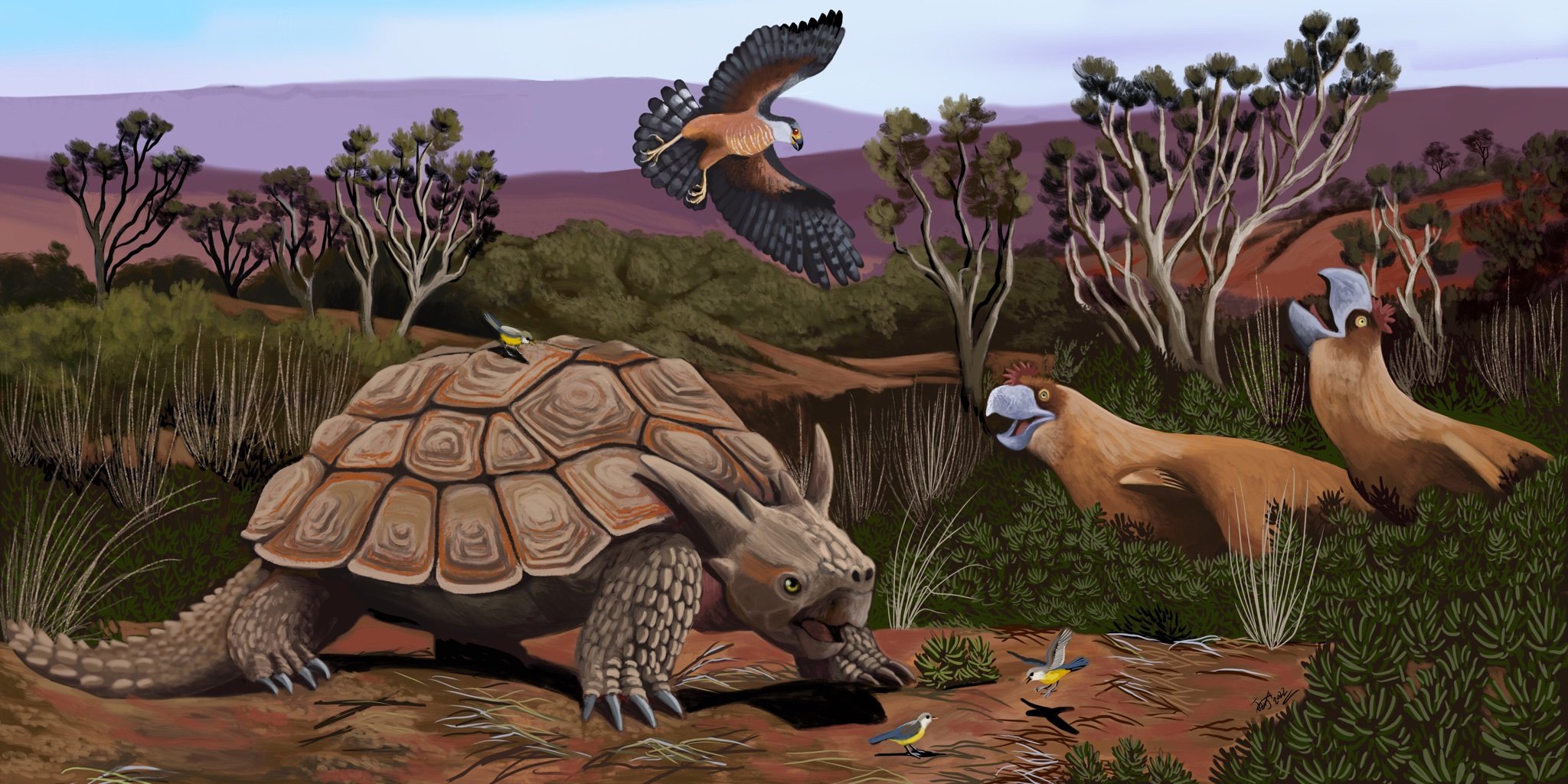The image is a detailed, realistic painting, possibly digital art, of a prehistoric scene featuring an array of unique animals and lush vegetation. Dominating the foreground is an enormous, primitive creature resembling a turtle, but with a body that is a hybrid between a crocodile and a turtle. This creature has a shell, long spiky tail, and a head that resembles a dinosaur’s, complete with two long protruding horns or ears. A small bird with blue and yellow feathers perches atop its shell.

To the right of this main creature, two large, four-legged animals with long beaks and yellow eyes are seen sitting on the ground. The one on the right appears to have its head thrown back, almost as if laughing. Just above this pair is a bush, and soaring in the sky above the scene is a large bird with bluish wings, a brown body, and a white head.

The background is filled with sparse green trees reminiscent of an African safari landscape, with hills and tall grass adding depth to the scene. Additionally, two small birds can be seen walking around on the ground, enhancing the prehistoric ambiance of the painting.